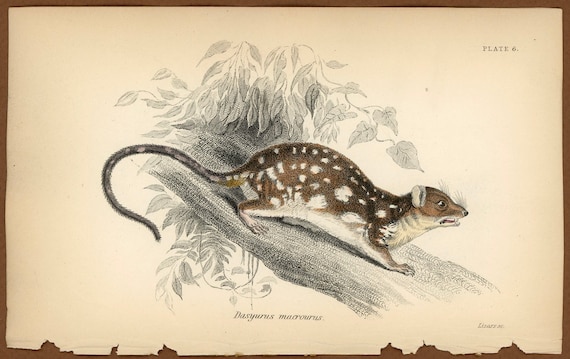This horizontally aligned, rectangular image appears to be an old print, possibly a lithograph or etching, resembling something you might find in an antique book. The image is bordered by a thin wooden brown frame with an ivory or light tan backing. The main subject, a small mammal facing to the right, is centrally placed. The animal, likely resembling a squirrel or gerbil, features a brown body with white patches on its back, a white underside, and a gray tail with white spots. Its right-side profile reveals beady eyes, a small ear, whiskers, and an open mouth that makes it look slightly angry. The creature is perched on a detailed black and white tree branch, surrounded by leaves of the same monochromatic tones. Faintly printed in fine text at the bottom, it appears to read "Desirius Macrorus" or something similar, while the upper right corner of the image is marked "Plate 6." The print itself suggests age, evident from its lightly beige, almost ripped paper texture.